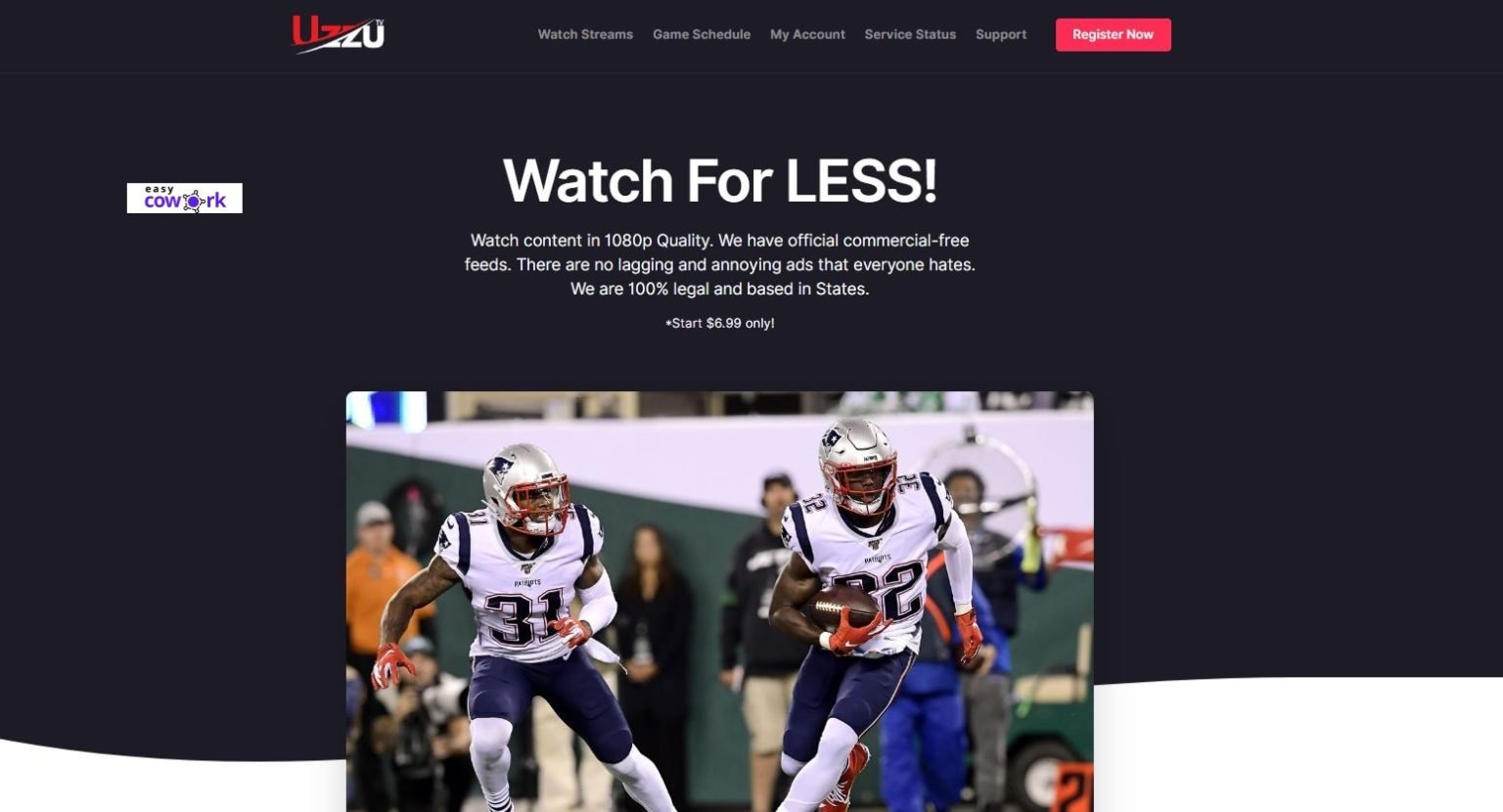In the center of the image, "Watch for Less!" is prominently displayed in white text, with the word "Less" in bold. Below that, the caption reads, "Watch content in 1080p quality. We offer official commercial-free feeds. Enjoy a smooth experience with no lag and no annoying ads. Our service is 100% legal and based in the United States. Start for only $6.99."

At the bottom of the image, there are two football players in action. The player on the left wears a silver helmet and a jersey numbered 31, complemented by football pants and white undershorts. The player on the right, similarly dressed with a silver helmet, sports a jersey numbered 32. He holds a football in his hand and appears poised to run, accentuated by his red football gloves. At the very top of the image is the text "UCI," inside a red rectangle with an option to "Register Now."